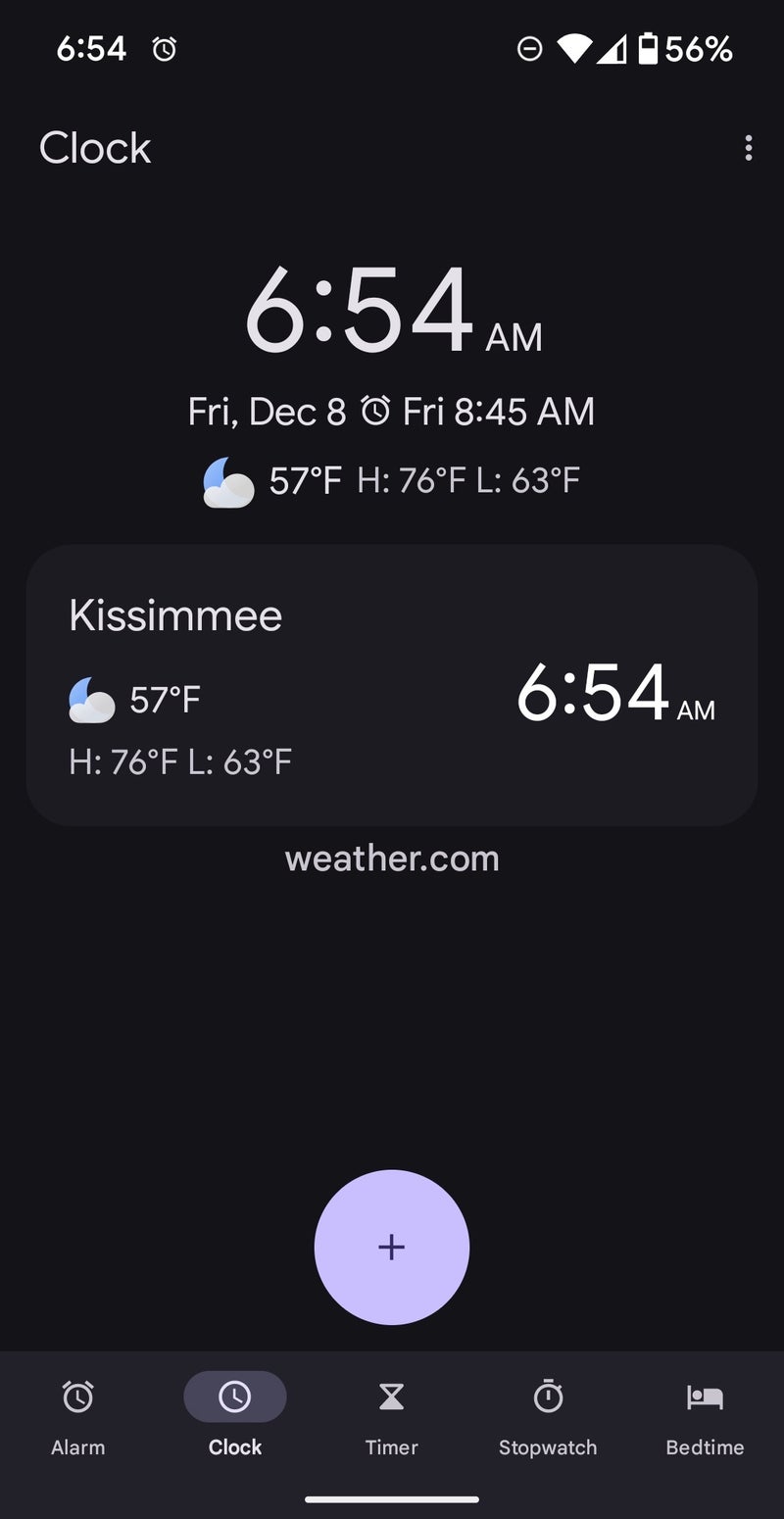A screenshot captured from a mobile device with a black background and white text displays detailed information. At the top left corner, the time is indicated as 6:54. On the top right, several icons are present, including a battery icon showing 56% charge. Centrally positioned, in a bold font, is the time displayed again as 6:54 P.A.M. Directly below this, the date is shown as "Friday, December 8th," alongside an alarm icon indicating an alarm set for 8:45 A.M. 

Further down, the weather forecast is displayed, followed by a name, "Casey Mee." The weather details are reiterated below the name, accompanied by the weather.com URL. At the very bottom of the screen, a lavender-colored circular icon with a plus sign is situated in the middle.